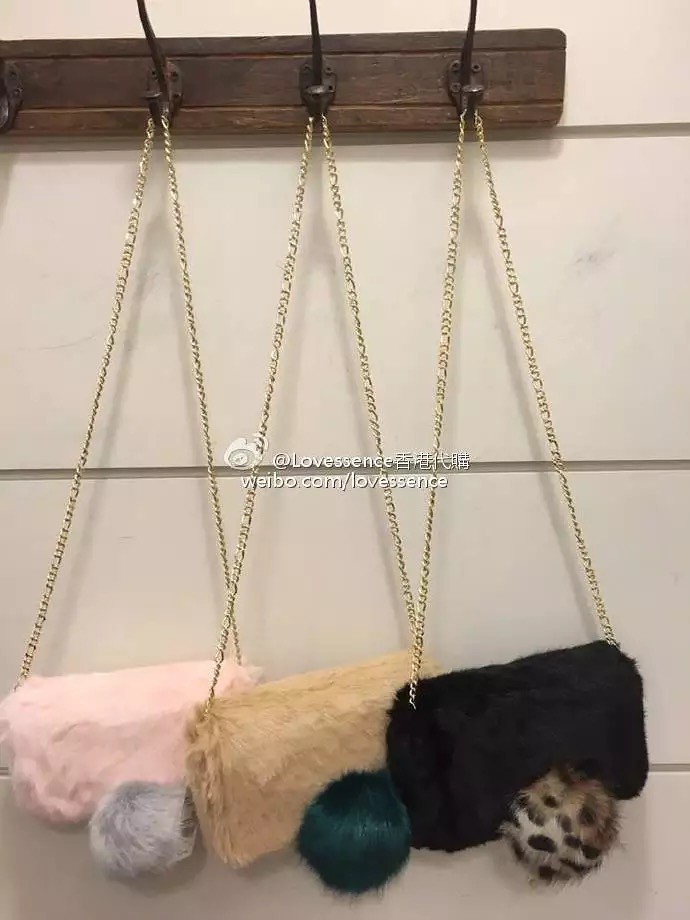This color photograph captures three small, rectangular coin purses with long gold chain handles, hanging from a wooden coat rack affixed to a white wall. The rack features four dark brown metal hooks, with each hook holding a purse of various colors and decorative pom-pom balls. From left to right, the purses are as follows: a fluffy pink purse with a gray pom-pom, a tan purse with a deep emerald green pom-pom, and a black purse adorned with a leopard-patterned pom-pom. The rack and the purses are the primary focus against the minimalist white background. Centered in the photo is a watermark reading "Love Essence at Weboo.com."